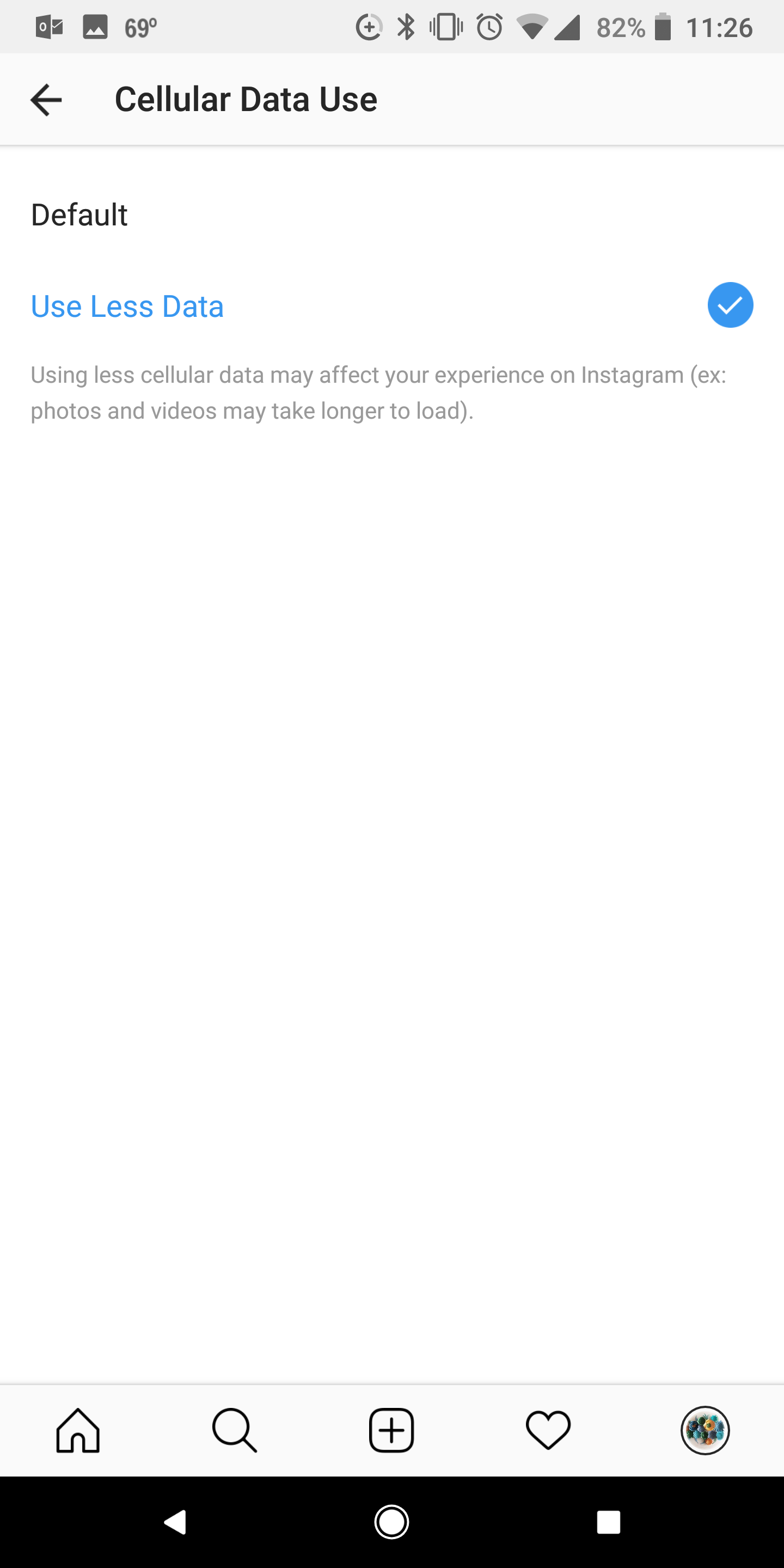A detailed caption for the image described:

---

The screen of a cell phone displays a settings page with distinctive elements. At the top, the status bar is shaded gray, showing the temperature as "69 degrees" accompanied by a degree symbol. A small black box features icons representing mountains and an envelope. Centrally positioned are time and status indicators: a half-circle black icon with a gray section and a plus sign in the middle, a cell phone outline, a clock, signal strength, and volume icons—all in black. The battery icon indicates "82%" with corresponding color fill.

The time reads "11:26". Below, a section labeled "Cellular Data Use" has a left-pointing black arrow. The background transitions to white, displaying the word "Default." Under this, the option "Use less data" is shown with a blue circle containing a white check mark to the right. An advisory note reads, "Using less cellular data may affect your experience on Instagram (example: photos and videos may take longer to load)."

The screen's background remains white, with a navigation bar at the bottom showing icons in black: an outline of a house, a magnifying glass for search, a square with a plus symbol, a heart outline, and a profile outline encircled with dots. The very bottom of the screen is black, featuring the navigation buttons in white—a triangle, a circle, and a square for back, home, and recent apps, respectively.